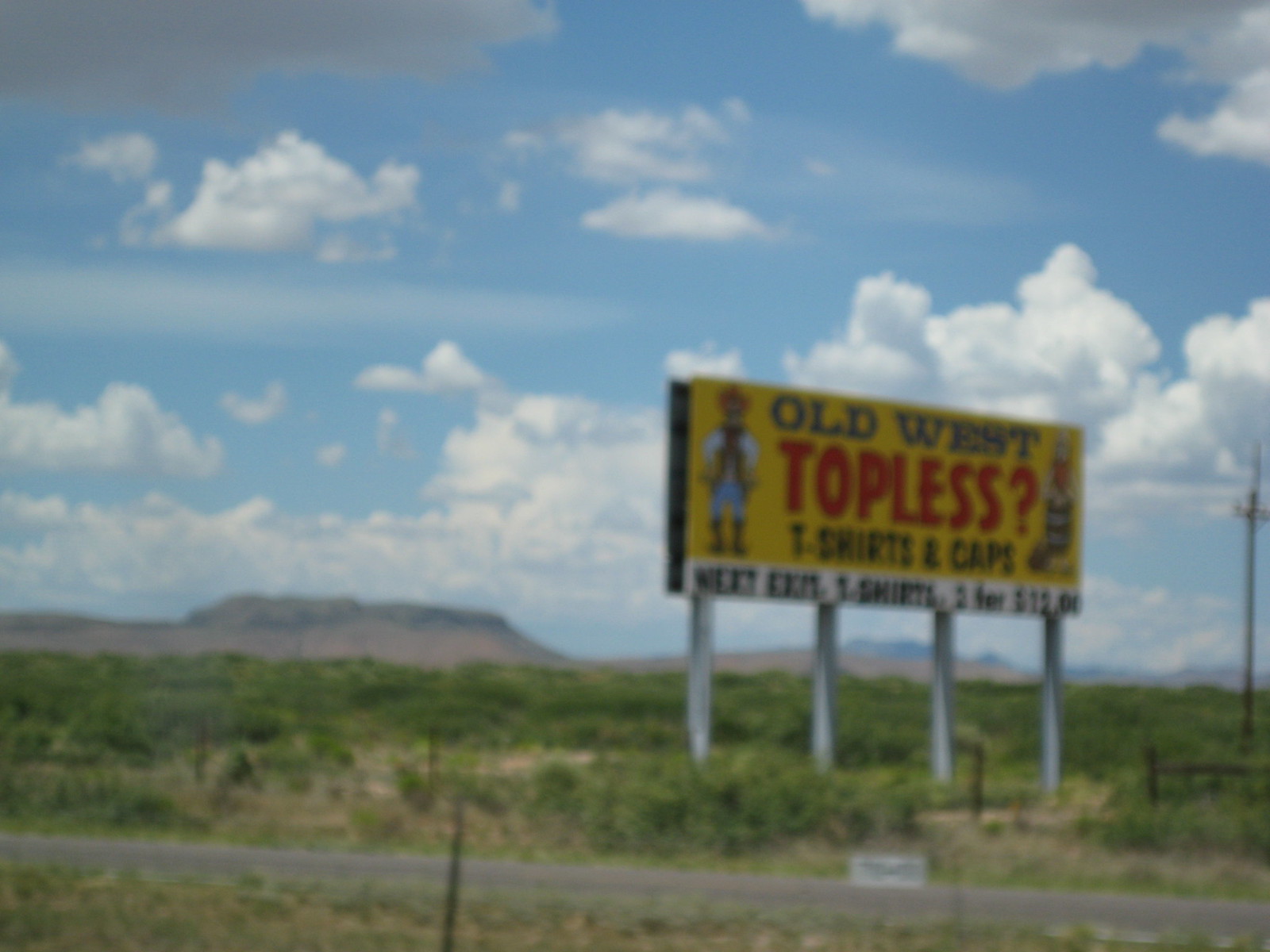The image depicts a blurry photograph taken from a moving vehicle on a highway, showcasing a large yellow billboard set against a remote desert landscape. The billboard, mounted on four gray posts, is prominently positioned alongside the road and features bold, attention-grabbing red and black text. The main headline in bright red letters reads, "Old West, topless?", with a question mark for emphasis. Below that, additional text advertises "T-shirts, caps, next exit" in black letters and a promotion stating "T-shirts: two for $15" in smaller writing on a white bar at the bottom of the sign. The billboard also includes illustrations possibly depicting cowboys or Western-themed characters flanking the word "topless." The scenic backdrop features a desert terrain with low green brush, plateaus or brown-colored mesa-type hills, and darker mountains in the far distance. The sky is a clear blue adorned with cumulus clouds, enhancing the openness and isolation of the setting. The entire scene is framed by a faint outline of an old-time fence and an adjacent dirt road running parallel to the highway.